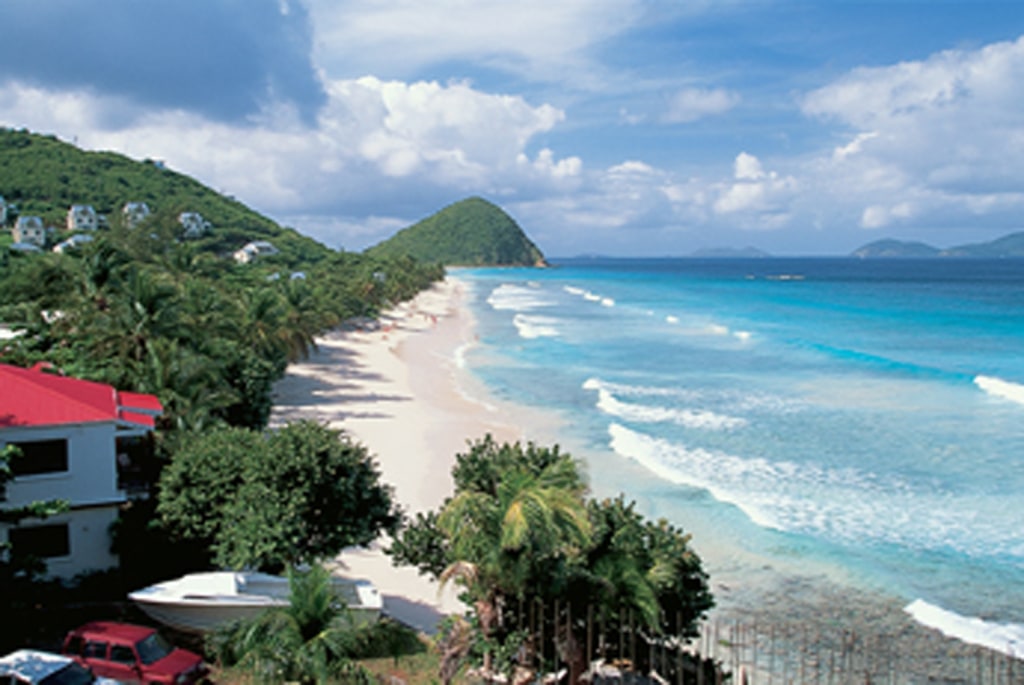In this photograph, we see an idyllic, tropical beach scene captured from an elevated perspective. The centerpiece of the image is a white sandy beach flanked by brilliantly blue ocean waters with gentle white-capped waves. Toward the horizon, a lush, green mountain rises dramatically, indicating another island in the distance. 

In the foreground, there is a two-story white house with a striking red roof, featuring large windows. Parked nearby, we can identify a white powerboat, a white SUV, and a red station wagon. 

The scene includes a notable contrast between natural and human-made elements: the dense greenery of the forest that stretches right to the beach's edge, interspersed with palm trees and primitive stone statues on a hillside. 

Adding to the atmospheric mood, thick masses of clouds hover over the top-left and top-right portions of the image, conveying a cloudy day. A wooden fence marks the transition from the built environment to the pristine beach. The photograph is a vivid portrayal of tranquil beauty, where verdant foliage meets the vibrant blues of the ocean.